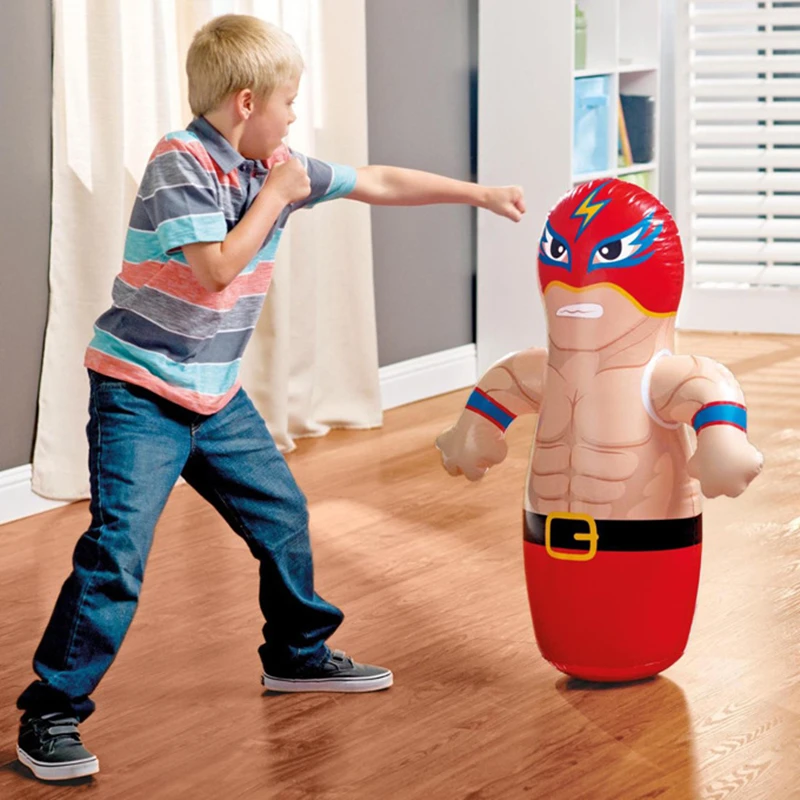In this square photograph, a young boy, approximately 10 or 11 years old with short blonde hair, stands poised on a hardwood floor in a home, preparing to punch a large inflatable doll designed to look like a cartoon wrestler. The boy is positioned on the left side of the image, facing right. He is wearing a short-sleeved polo shirt with gray, blue, light blue, orange stripes (separated by thin white stripes), blue jeans, and gray velcro sneakers with white soles. The boy's legs are spread wide, his left arm extended in a jab, and his right arm bent protectively in front of his chest. His determined expression complements his fighting pose.

The inflatable wrestler stands to the right, featuring a red luchador mask with a yellow lightning bolt on the forehead, a mean expression, muscular arms stretched out, and red bottoms with a black belt and gold buckle. This punching bag is weighted at the bottom, allowing it to bounce back after each hit.

The background reveals an interior room with white walls, white baseboard molding, and a hardwood floor. To the far right, there is a white bookshelf with various items, including some books, a blue box, and a green water bottle. Behind the inflatable doll, horizontal blinds cover a window, and part of a long off-white curtain is visible, adding a homely touch to the spirited scene.